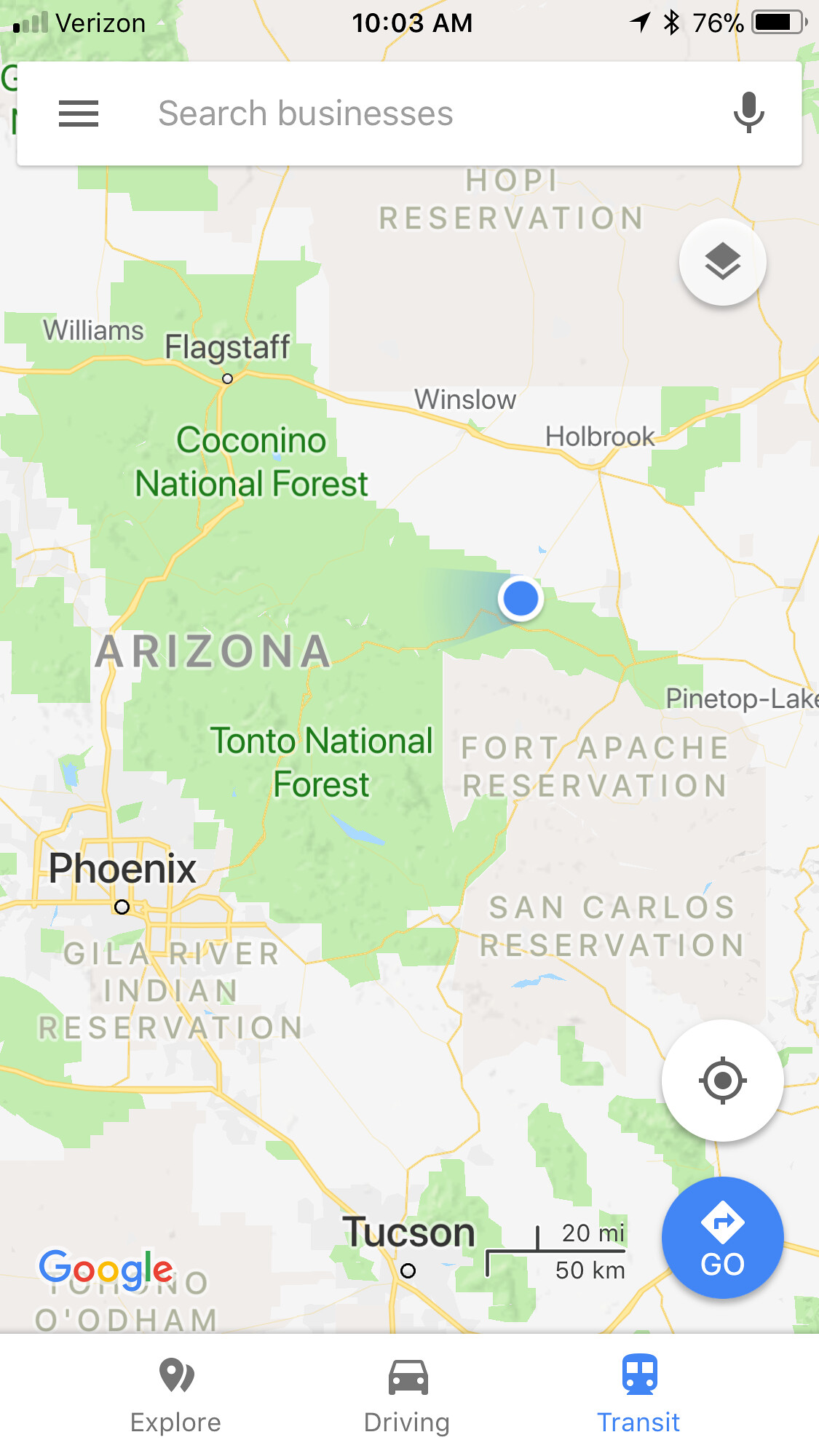The image depicts the screen of a smartphone, displaying a Google Maps interface. In the top left corner, the Verizon network name is visible along with signal strength bars. The upper right corner shows a battery indicator at 76% and the time reads 10:03 a.m. prominently at the center top. 

Beneath the time, there's a search bar labeled "Search for businesses" accompanied by a microphone button for voice search. The main portion of the screen is occupied by a detailed map of Arizona, featuring significant geographical and urban areas. The map highlights the Tonto National Forest and Coconino National Forest, with specific marked regions such as the Hopi Reservation, Phoenix, Gila River Indian Reservation, San Carlos Reservation, and Fort Apache Reservation. Tucson is indicated towards the bottom of the screen.

At the very bottom of the interface, there's an indicator bar showing distance markers of 20 miles and 50 kilometers. The Google Maps logo is displayed in the bottom left corner. The bottom right corner contains a circular button, presumably for locating the user's position, along with a goal icon. A blue highlight marks a specific area in Arizona, situated just to the upper left of the location labeled Pinetop-Lakeside, southwest of Holbrook, and south of Winslow. 

The navigation options include buttons labeled "Explore," "Driving," and "Transit" arranged at the bottom of the screen, providing various map views and navigation modes.